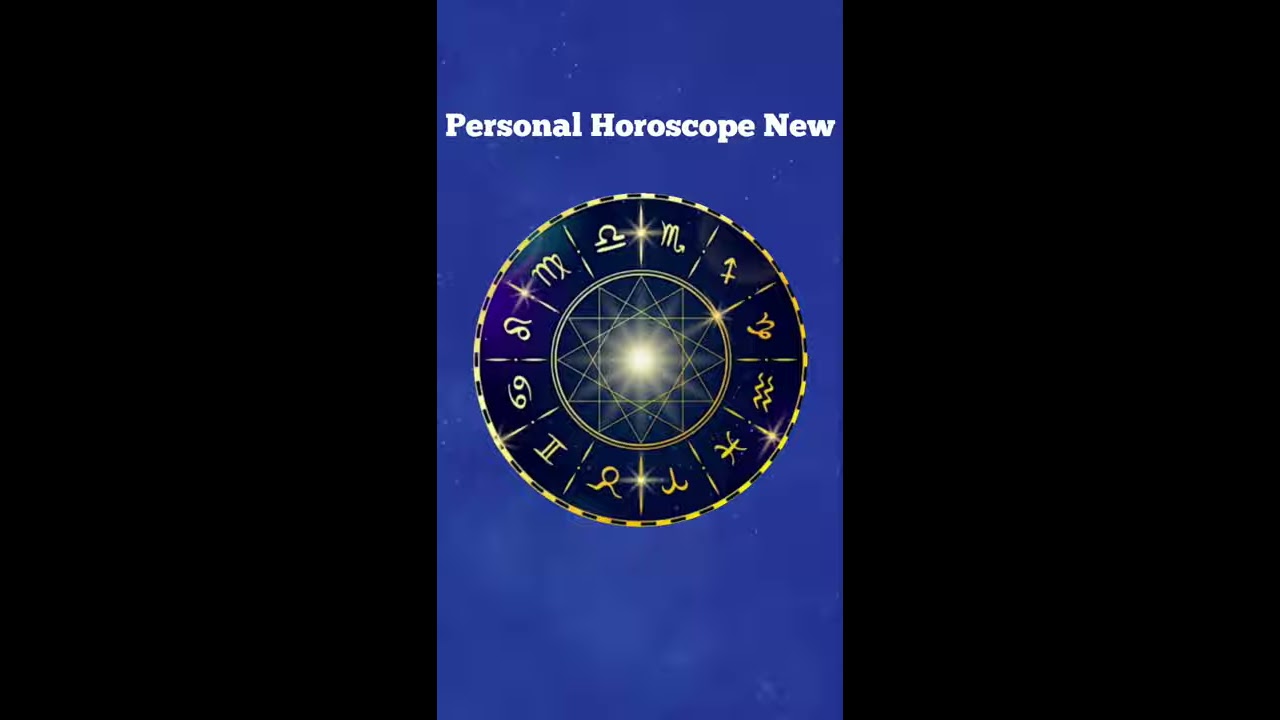This digital poster in portrait orientation showcases an astrological theme. At the top, in a bold serif font, white text reads "Personal Horoscope New," with the first letter of each word capitalized. The primary focus is a large, dark blue circle, centrally positioned against a lighter blue background speckled with faded stars, creating a celestial ambiance. Flanking the background are two vertical black strips that border the image.

The central circle is intricately detailed, divided into 12 segments by alternating long lines and dots, each segment containing a yellow zodiac symbol. The outer part of the circle, adorned with these yellow zodiac signs, encases a geometric pattern with 12 angles around a radiant sun depicted in gold at the center. This geometric design, combined with the astrological symbols, creates a striking visual representation of the zodiac wheel, giving the image a mystical and cosmic aesthetic.